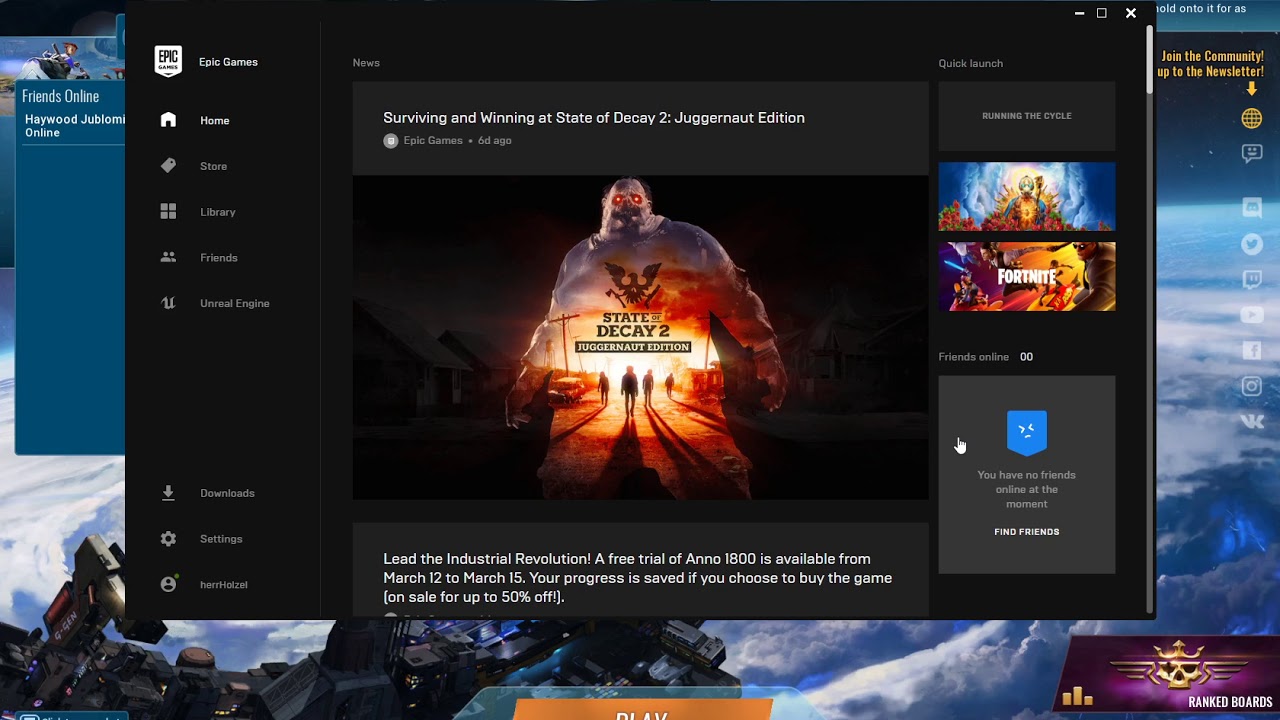A detailed screenshot captures the Epic Games application interface on its home page. The application is not accessed through a browser, as there's no browser heading on the window, but rather through a standalone app.

On the top left corner, the Epic Games logo is prominently displayed. Adjacent to this, a large vertical navigation bar lists various sections: Home, Store, Library, Friends, and Unreal Engine. Below a spaced divider, additional options such as Downloads and Settings are visible, along with the profile name "HERRHOLZEL," indicating the currently logged-in user.

The central area showcases the cover image for "State of Decay 2 Juggernaut Edition," featuring a visually striking depiction of an undead creature with a sunset within its silhouette. The apocalyptic backdrop further enhances the image's eerie atmosphere, with humanoid figures advancing in the foreground.

On the right sidebar, thumbnails for other popular games such as Fortnite are displayed. In the bottom right corner, a friends list denotes that there are currently no friends connected, accompanied by a prompt to find friends and an icon of a blue face with a grimacing expression.